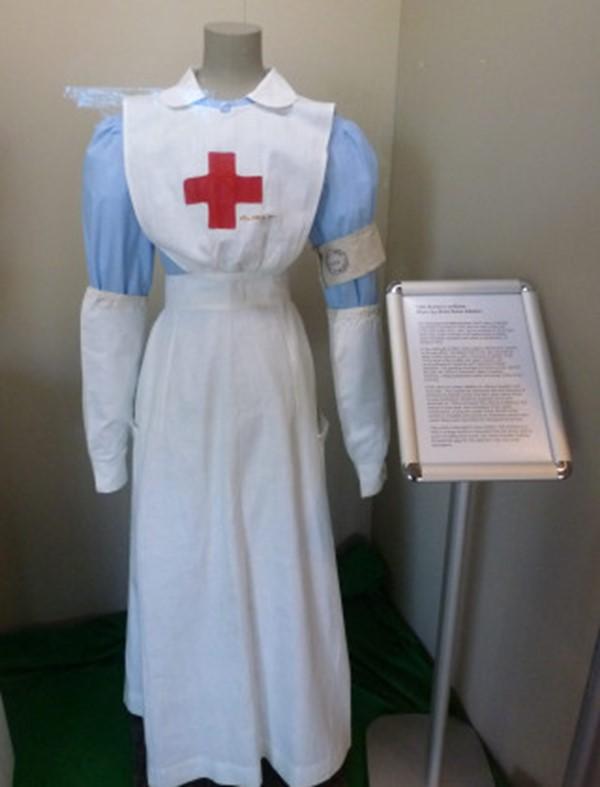The photograph captures a museum exhibit featuring a headless mannequin dressed in a historical nurse's uniform. The mannequin stands in a white-walled corner, showcasing an intricate outfit composed of several layers. The base layer is a light blue dress, noticeable around the shoulders and partially down the arms. Over this, the mannequin dons a long, white smock that reaches from the neck to the floor, resembling a full-length skirt with numerous folds and a prominent white bib at the top. The smock features a red cross emblem prominently displayed at the center of the chest. Both arms of the mannequin are wrapped in white cloths up to the elbows, giving the appearance of gloves that cover the forearms, though there are no visible hands or further details.

Next to the mannequin, a tall placard on a silver stand provides detailed information about the exhibit, though the text remains unreadable from the photograph. The placard is about waist-high when compared to the mannequin, emphasizing its informative role in the display. The entire setup, with its detailed attire and accompanying explanation, clearly situates the mannequin as a representation of a nurse, complete with historically significant uniform elements.